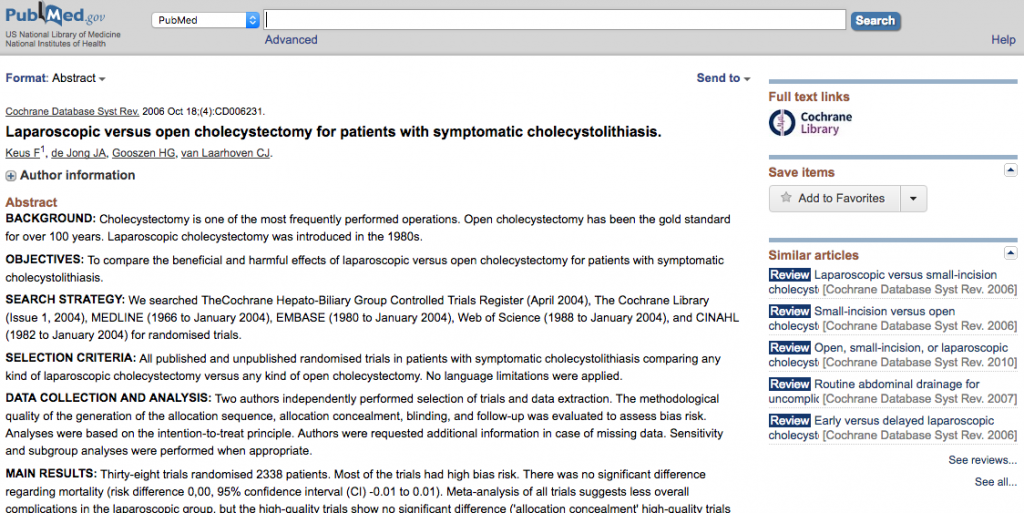The image captures a screenshot of an older, text-heavy website interface, identified as pubmed.gov. The webpage features a plain white background with a gray search bar at the top. The central content of the page is an academic article titled "Laparoscopic versus open cholecystectomy for patients with symptomatic cholelithiasis," written by medical researchers. On the right side of the page is a sidebar with a "Full Text Links" section highlighted in brown text, along with a reference to the Cochrane Library, suggesting where the article might be stored. Additionally, the sidebar includes similar articles. There is a help link at the top right corner of the page, and the search bar at the top includes a dropdown menu for different types of searches.